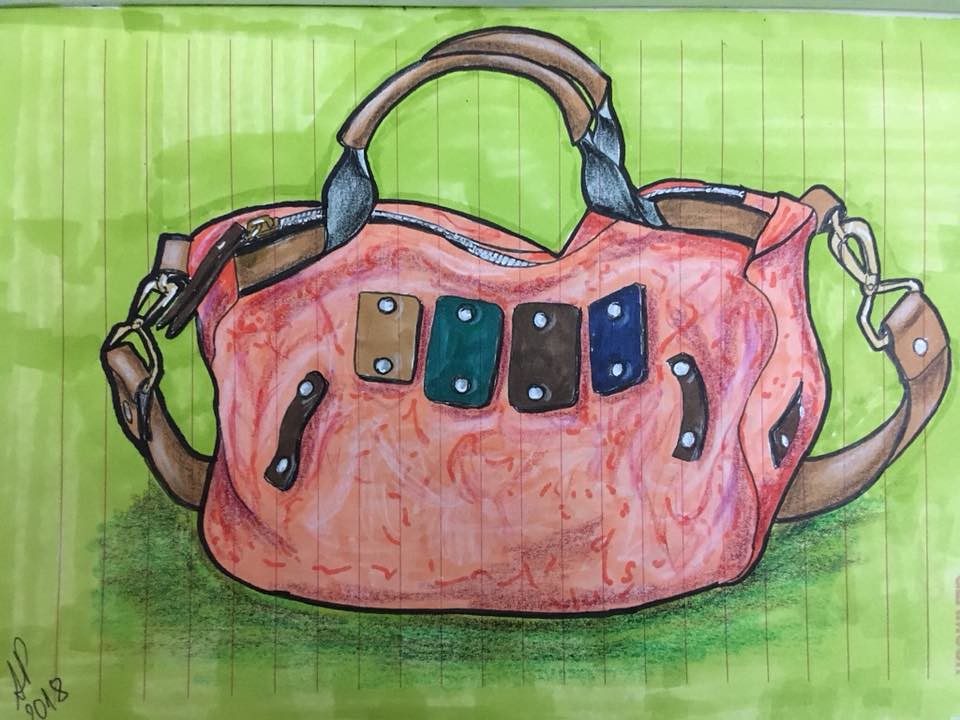This meticulously crafted drawing, likely created with colored pencils, markers, or pastels, is set on what appears to be ordinary notebook paper with vertically oriented lines. The background is thoughtfully sketched in various shades of green, including lime, darker green, and olive tones. At the center of the artwork is a striking depiction of a women's handbag, predominantly rendered in a vivid reddish hue. The front of the handbag features four decorative vertical strips in tan, aqua blue, dark blue, and dark brown. The bag is detailed with a top zipper and handles, along with a removable shoulder strap attached by hooks on either side. The artist has rendered these elements with exceptional precision, showcasing a visually appealing and highly detailed piece.